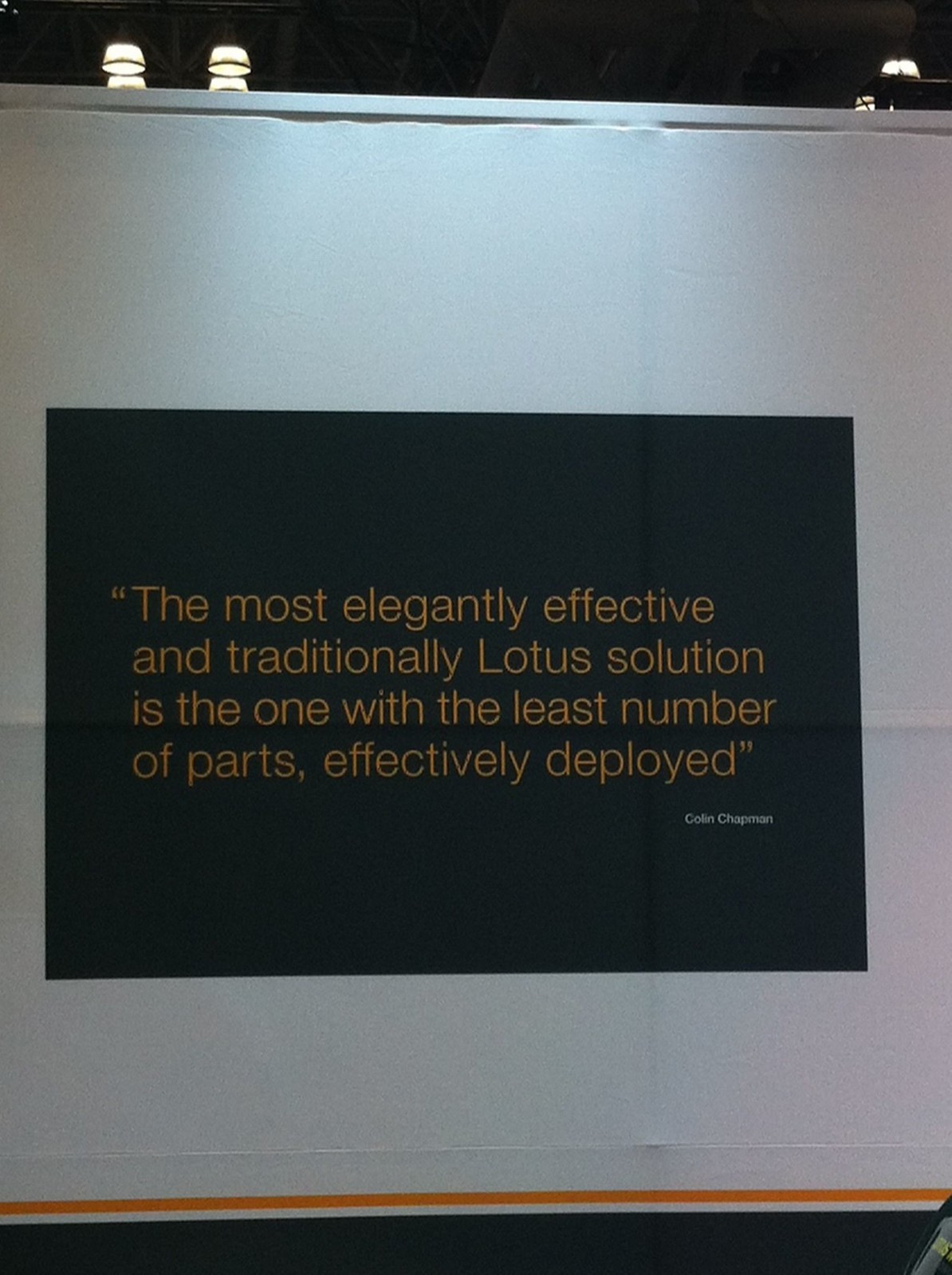The image captures a white wall illuminated from above, lending a subtle brightness to its top section while casting shadows towards the corners and bottom. Central to the wall is a black rectangular text box with visible creases, suggesting it may be painted on or part of a fold-out display. Within this black box, a quote is elegantly inscribed in gold lettering: "The most elegantly effective and traditionally Lotus solution is the one with the least number of parts effectively deployed." At the bottom right of the text box, the quote is attributed to Colin Chapman, with his name written in white. Overhead, a couple of lights and a black upper section of the wall or ceiling are faintly visible, though the ceiling itself remains out of the frame.